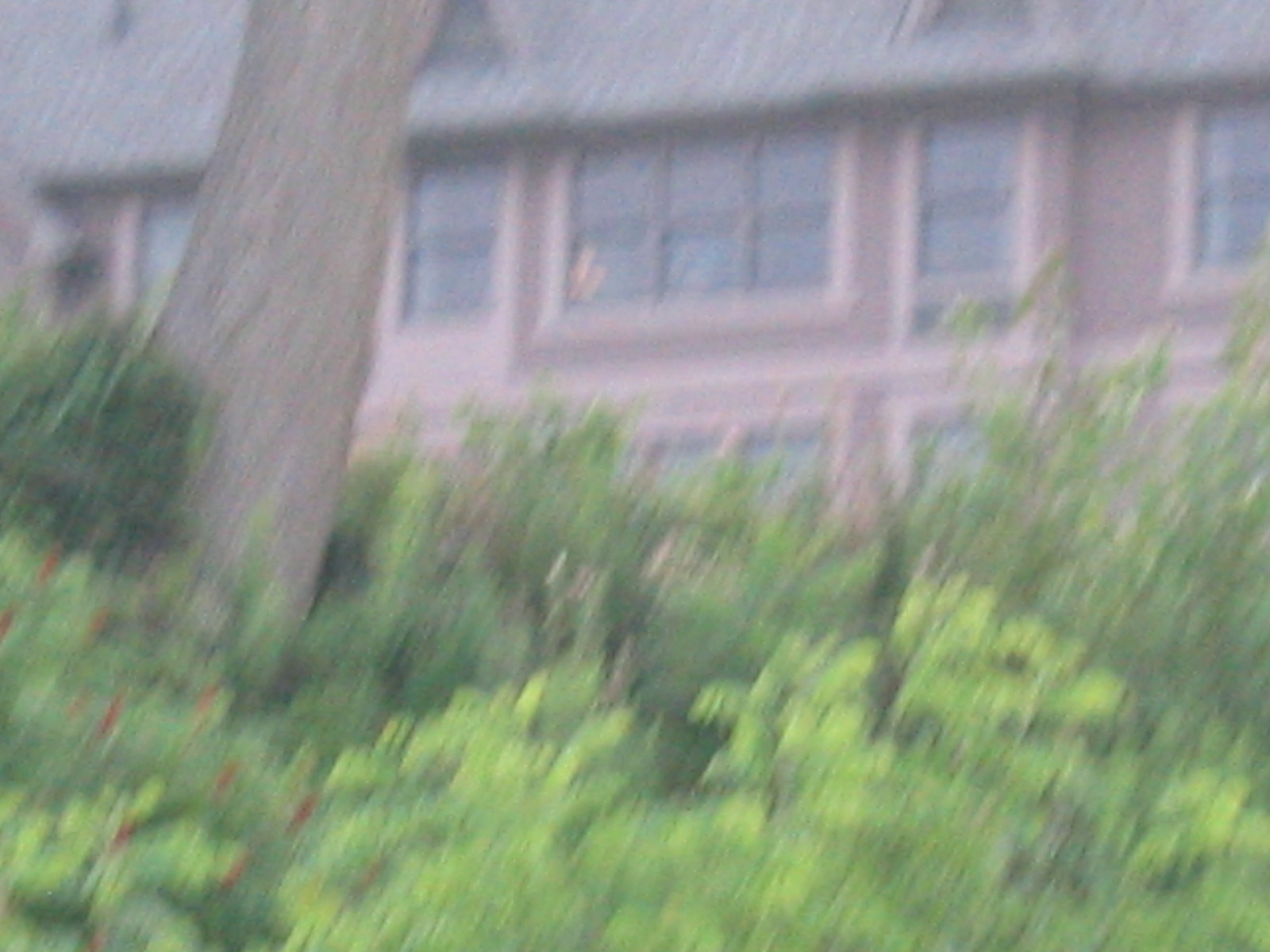The image depicts a very blurry side shot of a large building, possibly a mansion, characterized by its distinct architectural elements and dense surroundings. The building, appearing to be mauve or slightly pinkish in color, features several large windows on the second floor, through which a light can be seen glowing, though no people are visible. On the top center of its slanted grayish roof are two triangular windows, enhancing its grand appearance. The lower part of the building is almost completely obscured by lush green foliage and dense clusters of plants, among which is a large tree trunk that extends from the far left of the frame, angling to the right and reaching up out of view. Despite the overall blurriness, which suggests it may have been taken hurriedly or without focus, subtle details like the texture of the foliage and the window structures are noticeable.